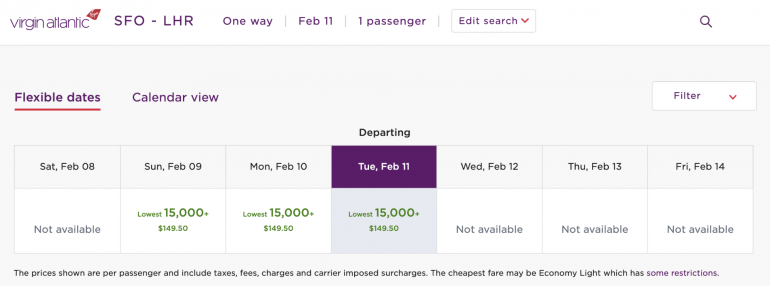In the top part of the image, the background is white. On the left-hand side, "Virgin Atlantic" is written in purple. Adjacent to this, there is a red diamond shape with some white print inside it that is not clearly visible. 

Next to the red diamond, "SFO-LHR" is displayed in purple, capital letters, indicating the route from San Francisco to London Heathrow. To the right, it says "one way" in purple. Following this, there is a vertical gray line, beneath which it reads "Subway 11." Coming after another gray line are the words "one passenger."

Further down is a white rectangular box with a gray border that contains the text "at his search" in purple. An arrow pointing down in red is at the end of the text. To the far left, there is a gray rectangle with the words "flexible dates" written in purple and underlined in red. Next to this, it says "calendar view."

Below this section, the specific dates and availability for flights are listed:
- "SAT February 08" is shown in black with a notation "not available."
- For "Sunday, February 09," it says "lowest" with a price of "$15,000 plus $149.57," highlighted in green.
- Similar information is repeated for "Monday, February 10," "Tuesday, February 11," and "Wednesday, February 12."
- Dates for "Thursday, February 13" and "Friday, February 14" both indicate "not available."

This detailed layout appears to outline flight options and their availability for a specified route.